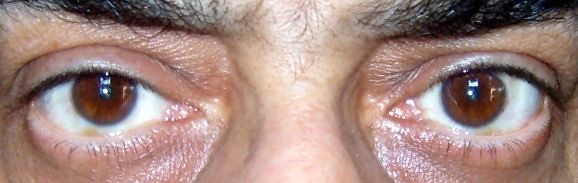The image is a close-up of a man's eyes and the bridge of his nose, emphasizing his dark, furrowed eyebrows and hazel brown eyes with clear whites. His medium tan skin features slight signs of swelling around his eyes and dark circles, giving him a somewhat concerned look. His eyebrows are thick but not well-maintained, with a few stray hairs between them. The man's eyes appear wide and intent, and despite having thin eyelashes, the gradient in his hazel brown eyes—from a near-black pupil outward to a lighter brown—stands out. There are a couple of blood spots in his eyes, enhancing the intensity of his gaze.